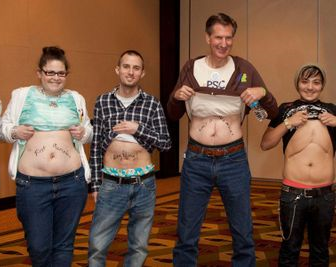In a spacious room with large walls and carpeted floors, a group of four individuals stands side by side, all lifting their shirts to expose their stomachs. On the far left is a woman with black hair styled in an updo, wearing glasses and a green and white shirt paired with blue jeans. She has black writing around her belly button. Next to her is a man dressed in a white and blue plaid shirt, similarly exposing his stomach, which also displays some writing. The tallest man stands to his right, sporting brown hair and a brown shirt over a white undershirt, with black writing above his belly button. On the far right is a young girl, wearing a cap and smiling, revealing her entire chest. She appears to be a transgender person with visible hair on her chest. The exposed stomachs of the group prominently display markings, which include tattoos and scars.